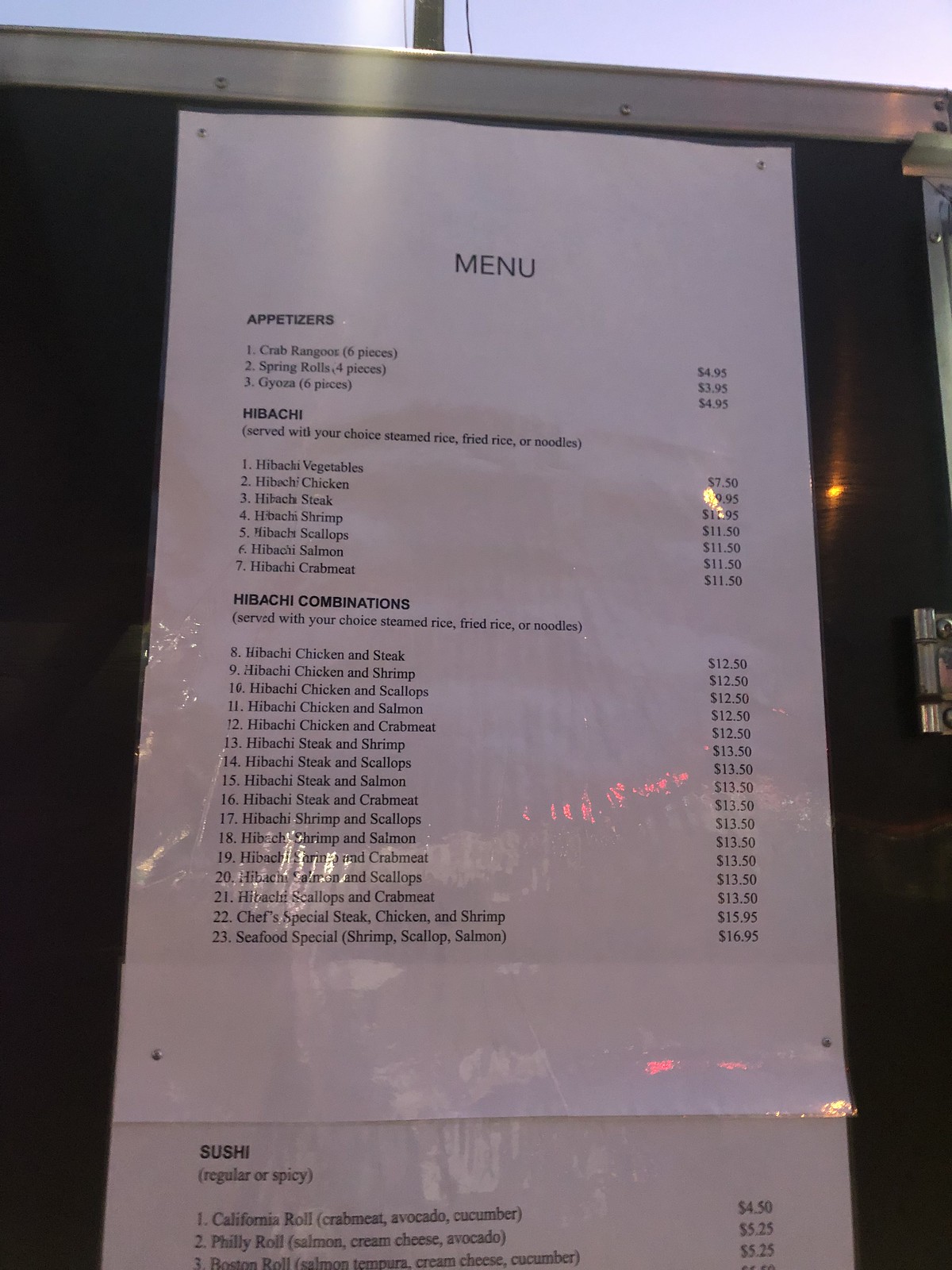The image features a simple, yet functional, laminated menu of a Japanese restaurant affixed to a glossy, black door. Three laminated sheets are pinned vertically one above the other using silver tacks, clearly displaying the restaurant’s offerings. The hinge of the door is visible to the left, adding a touch of context to the setting.

At the top of the menu, "Menu" is prominently displayed in large font. The menu is divided into several main sections: Appetizers, Hibachi, Hibachi Combinations, and Sushi. Each section is neatly listed on the left side, numbered and accompanied by corresponding prices. For instance, the appetizers are numbered 1 to 3, Hibachi dishes range from 1 to 7, and Hibachi Combinations span from numbers 8 to 23. An example item is "Hibachi Chicken and Steak" which is priced at $12.50.

The overall presentation of the menu is straightforward and clear, providing a succinct overview of the dishes available in this Japanese eatery.